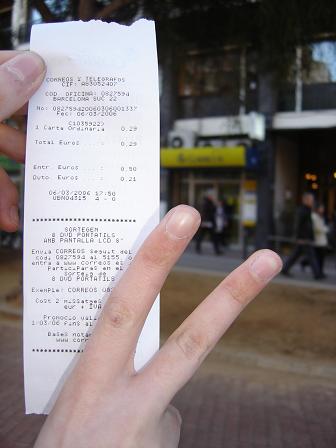In this photograph, a person is holding a black-and-white receipt on the left side of the image. The receipt appears to be for various computer and technology products and services, although the small writing makes the itemized list difficult to read. Positioned in the middle of the picture, another hand is visible, flashing a peace sign with two fingers in front of the receipt. The backdrop reveals a bustling cityscape with several buildings, each featuring numerous windows mostly situated towards the top. These buildings also have signage; one notable sign is rectangular and yellow with dark blue writing. The scene is lively with groups of pedestrians walking along the sidewalks, some likely entering or exiting the storefronts in the area.